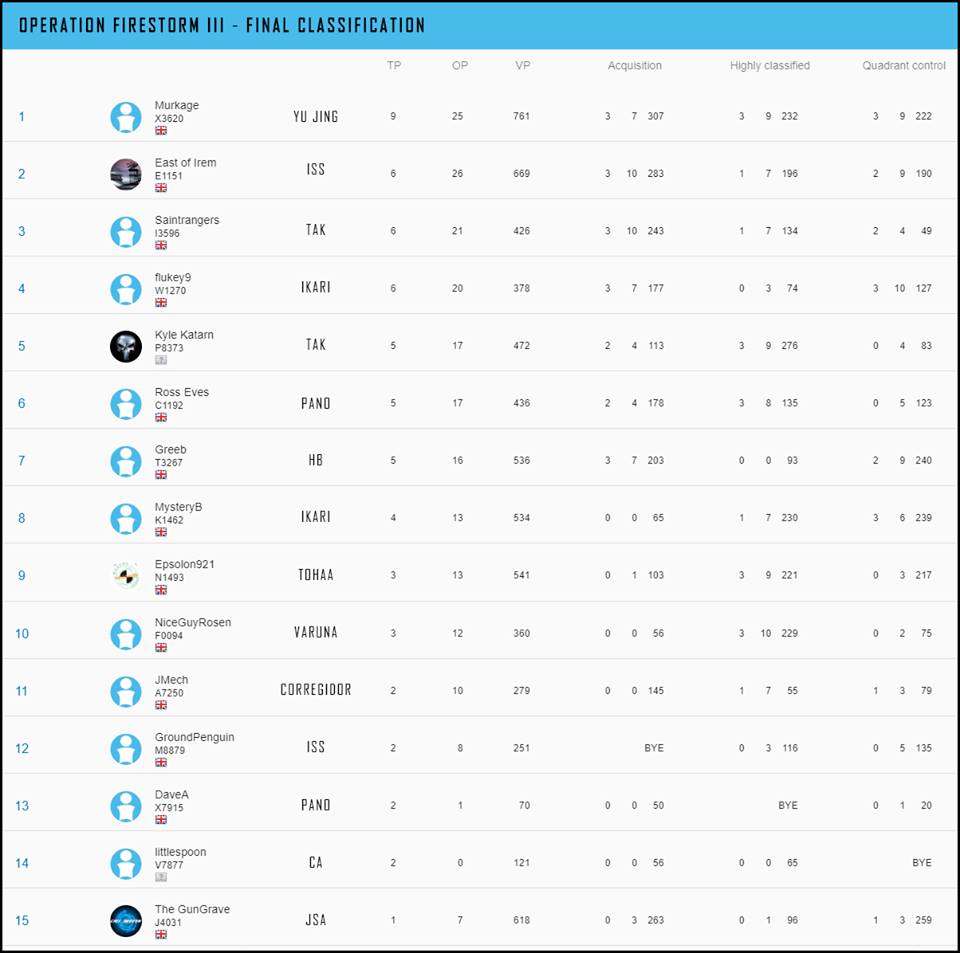This image displays the final classification for "Operation Firestorm 3," showcasing the rankings of 15 participants. The listed users are: Markage, East of IREM, St. Rangers, Fluky9, Kyle Katarn, Ross Eves, Grebe, MysteryBee, Epsilon921, NiceGuyRosen, Jmech, GroundPenguin, DaveA, Littlespoon, and TheGunGrave. The majority of these users appear to be associated with a faction or country symbolized by a red cross.

Additionally, there is a separate list of names that likely represent different factions or teams involved in the operation: Yujing, ISS, TAK, Ikari, TAK, Pano, HB, Ikari, Toha, Varuna, Corregidor, ISS, Pano, CA, and JSA.

The classification system includes several categories with numerical values assigned: TP (Tournament Points), OP (Objective Points), VP (Victory Points), Acquisition, Highly Classified, and Quadrant Control. This detailed breakdown suggests that the image is related to a structured competitive event, potentially involving strategic gameplay, where participants are ranked based on their performance across various scenarios.